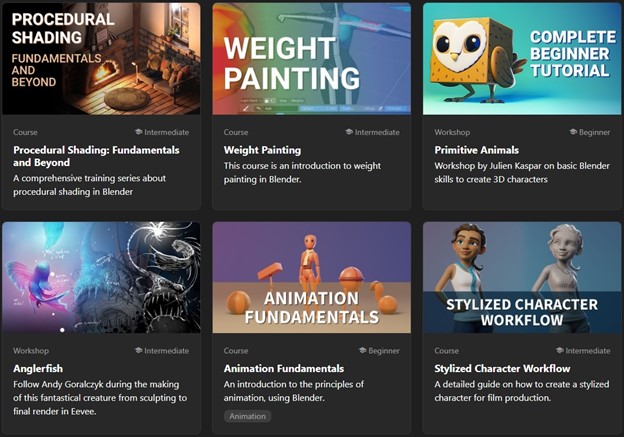This screenshot displays an unidentified platform lacking specific website details. The page features a black background with six distinct square icons, each representing a different course or workshop. The items are as follows: 

1. **Procedural Sanding** - Likely a detailed workshop or course focused on procedural texturing techniques.
2. **Weight Painting** - This seems to be a course centered on weight painting, possibly for 3D models.
3. **Complete Beginner Tutorial** - Designed for novices, this is probably an introductory course covering basic principles.
4. **Anglerfish** - This could be a specialized workshop or course, probably focusing on modeling or animating an anglerfish.
5. **Animation Fundamentals** - A course likely covering the basics of animation.
6. **Stylized Character Workflow** - This appears to be a workshop or course discussing the process of creating stylized characters.

Each item has a corresponding label indicating whether it is a workshop or course, suggesting that these educational resources can be enrolled in or completed online.